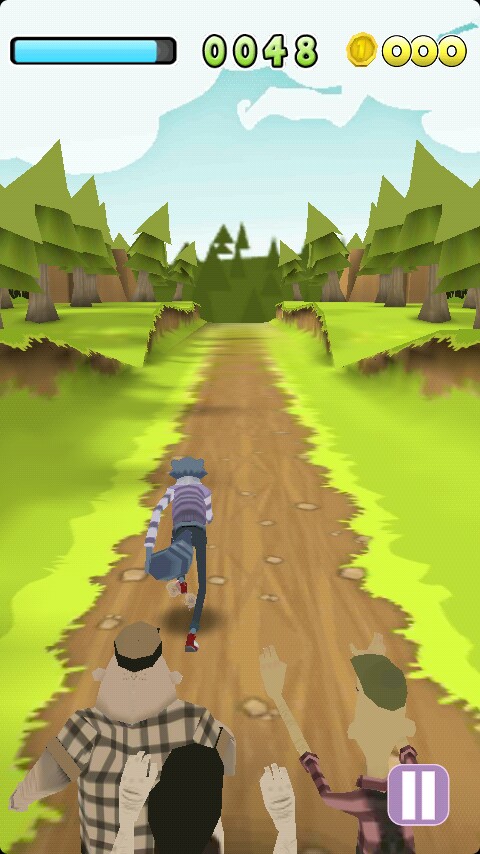This screenshot captures a scene from a mobile game, presenting a third-person perspective behind the player character who is running along a central path. The path, primarily brown, is interspersed with light brown speckled patterns along its edges. Flanking the path on both sides, there is flat green grass that gradually ascends to create raised embankments. These embankments are populated with lush green trees, each adorned with sturdy brown trunks. The image offers a vibrant and immersive view of the game's environment, highlighting the natural elements that frame the player’s journey.